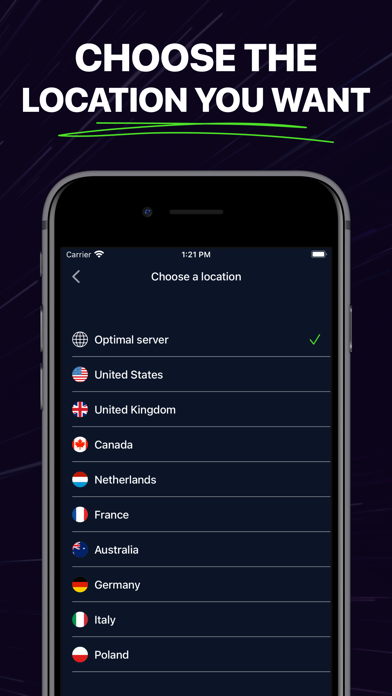In this image, we see a photograph of a smartphone, providing a detailed view of its screen and front-facing features. At the top center of the image, bold white text reads, "Choose the location you want." Directly beneath this text are three green lines. The main focal point is the smartphone itself, presented in a frontal view, capturing detailed elements.

At the top of the phone, we notice a circular, highly reflective front camera, situated slightly to the left. To its right, there is a light gray, rectangular bar. Moving to the actual phone screen, the top right corner displays a white battery icon. Centered at the top, the time is shown as "1:21 PM." On the top left, the word "Carrier" is displayed, followed by a fully filled Wi-Fi icon.

Below the time, in large text, it says "Choose a location." Various location options are listed on the left side of the phone screen, creating a vertical menu. These options include: Optimal Server, United States, United Kingdom, Canada, Netherlands, France, Australia, Germany, Italy, and Poland. Each location is clearly visible, contributing to the functionality and user interface of the phone's screen.